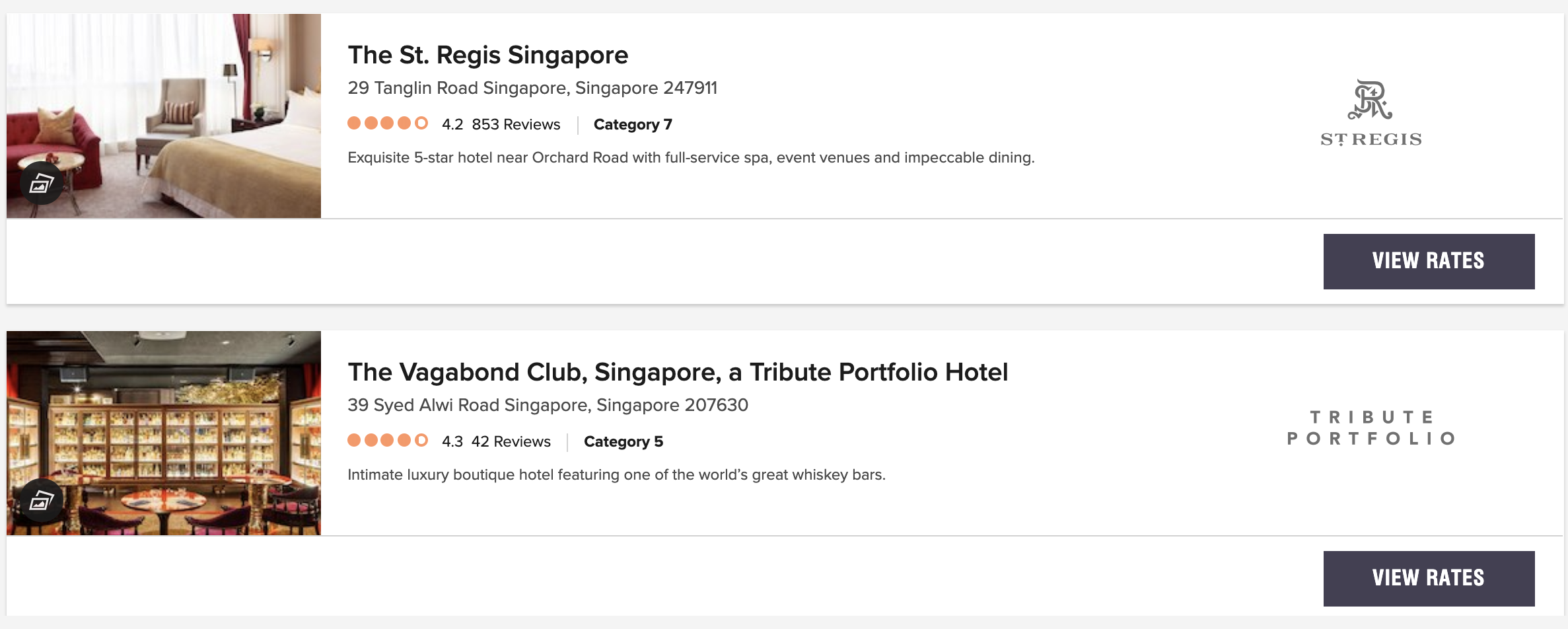This image depicts a travel booking website featuring hotel options without individual headers or detailed navigation. Displayed prominently are two hotel selections, each with accompanying photographs and descriptions.

On the left, the first hotel option showcases a photograph of a spacious bedroom. This room includes a large window allowing natural light to flood in, a striking red couch, a king-size bed, and a comfortable large chair paired with an ottoman. Directly below this individual shot, there is another image that appears to depict a cafe or a large bar, complete with refrigerator units likely containing various food options.

The description next to this imagery presents the St. Regis Hotel in Singapore, located at 29 Tanglin Road, Singapore, Singapore, 247911. The hotel boasts a rating represented by 4 out of 5 orange circles and has a review score of 4.2 based on 853 reviews. It is classified as a Category 7 hotel, offering an exquisite 5-star experience near Orchard Road, featuring a full-service spa, event venues, and impeccable dining options. The hotel's logo, an intertwined 'STR', and a "View Rates" button are situated to the right of the descriptive text.

Below this option, the second selection is the Vagabond Club, Singapore, a Tribute Portfolio Hotel. The photograph linked with this listing potentially represents one of the hotel's highlights: a renowned whiskey bar, indicating an intimate luxury boutique hotel atmosphere. The Vagabond Club has garnered a 4.3 rating with 42 reviews. The description mentions the hotel's intimate luxury and unique offerings. The logo and a "View Rates" button are likewise presented, with the hotel's address listed beneath its name.